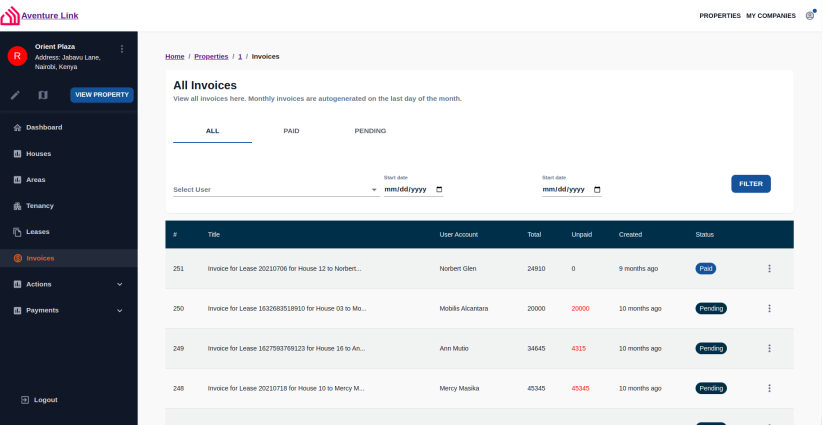This image displays a detailed web page layout. On the top-left corner, there is a distinctive logo featuring a house silhouette with smaller red stacks behind it, accompanied by the text "AdventureLink" in purple hyperlink style and underlined.

Below the logo, a dark blue vertical rectangle spans the length of the page, containing white text and a red circle with a white 'R' inside. The text reads "Orient Plaza, O-R-I-E-N-T Plaza," followed by the address "J-A-V-A-Y-U Lane, N-A-I-R-O-B-I, Kenya (Nairobi, Kenya)." This section also includes icons: a pencil silhouette, a bent square, and a dark blue "View Property" button with white text.

The side menu features several options, each with corresponding icons:
1. A house icon labeled "Dashboard."
2. A graph-filled square labeled "Houses."
3. Another square labeled "Areas."
4. Boxes resembling money labeled "Tertiary."
5. Two pieces of paper labeled "Leases."

An orange-highlighted item, indicating it's selected, displays an orange dollar sign in a circle and reads "Invoices." Additional menu items include:
- A graph-filled square labeled "Actions" with a dropdown on the right.
- Another similar square labeled "Payments."

The main content area is white, topped with purple tabs:
- "Home" with a black line.
- "Properties" with a black line.
- A combination of a numeral one and backslash.
- A blue "Invoices" tab.

On the top right, the navigation options include "Properties," "My," "Companies," and a bold, black "All Invoices," with "All" underlined and "Paid" and "Pending" beside it. There are sorting options like "Select User," "Select Date," and "Start Date" on the right side, followed by a list of payments at the bottom.